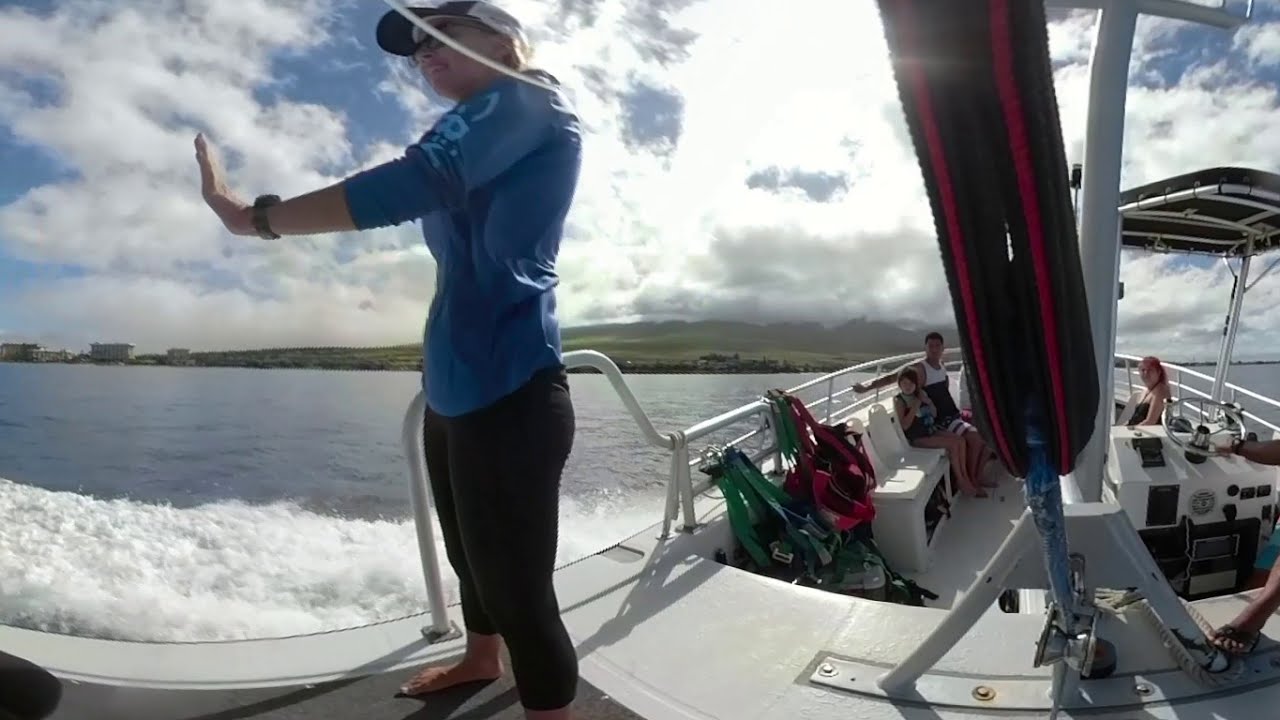In this vibrant and sunny image, a white motorboat cruises through the water, leaving a wake behind and revealing scenic, mountainous landscapes in the far distance beneath a bright blue sky dotted with fluffy white clouds. The boat's occupants include a diverse group of five people. At the center of the image stands a barefoot white woman, adorned in a black and white baseball hat, black sunglasses, a black watch on her left wrist, a long-sleeved blue top, and black pants. She waves her hand in the air, gazing off to the left. On the right side of the boat, a dark-skinned arm grasps the steering wheel, hinting at the person navigating the vessel. Nearby, a young boy with short brown hair wears a lifejacket, accompanied by an older man, likely his father, both of whom appear to be of Asian descent. They both don casual summer outfits. In the back, another woman with her red hair tied into a ponytail sits calmly, dressed in a black top. All individuals in the scene are barefoot, adding to the relaxed and carefree atmosphere on this lovely boat ride.